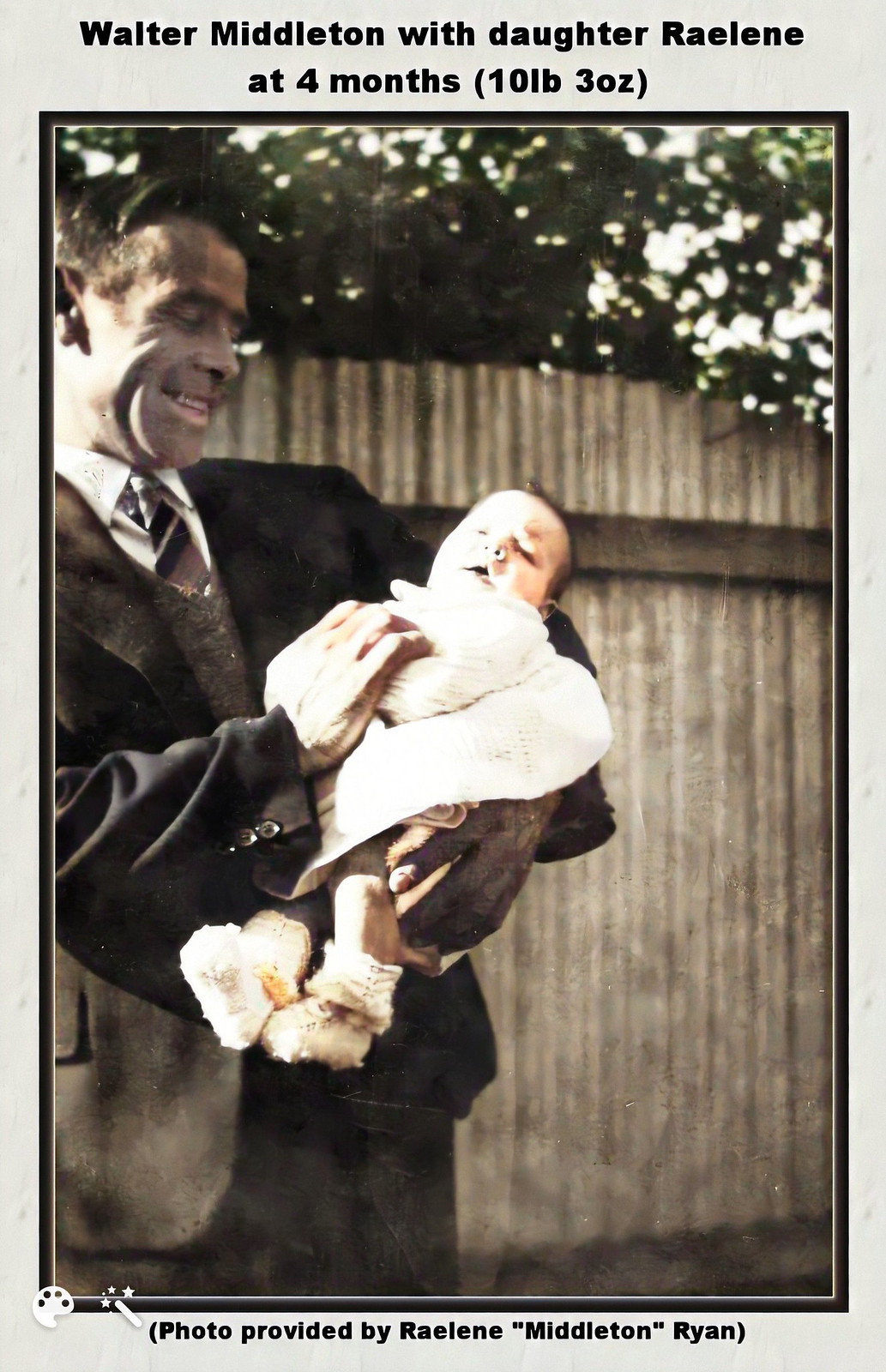This photograph depicts Walter Middleton proudly holding his daughter Raylene when she was four months old, weighing ten pounds and three ounces. The image, which is taller than it is wide, has been given a thin black border and an outer, wider gray border. At the top of the gray border, the text reads: "Walter Middleton with daughter Raylene at four months, 10 pounds, 3 ounces," and at the bottom it notes, "photo provided by Raylene Middleton Ryan."

Walter is dressed in a distinguished three-piece suit and is smiling warmly at his daughter. Raylene is snugly wrapped in a white blanket and wearing little white boots. The sunlight is illuminating the scene from the top left corner, causing Raylene to turn her face slightly away, with her mouth open and a small tuft of hair visible.

In the background, a tall wooden fence suggests a backyard or driveway setting, with green trees or bushes peeking over the fence, adding a natural and cozy element to the picture. Additionally, the lower left-hand corner of the photograph features an artist palette emoji and a magician's wand emoji with three stars around it, adding a whimsical touch to the presentation of this cherished memory.